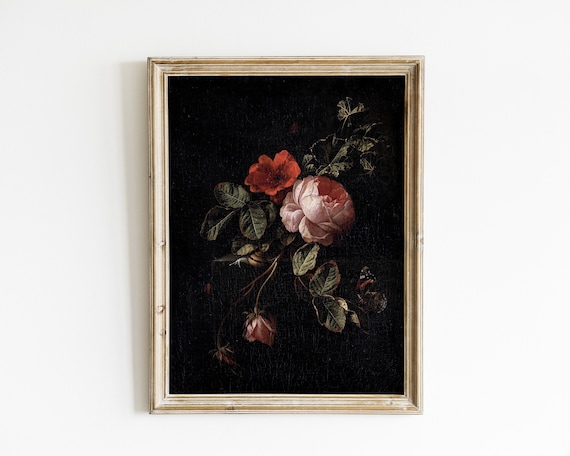This image captures a painting mounted on a white wall, encased in a light gold frame. The painting itself is set against a solid, jet black canvas, which exudes a somewhat melancholy, yet strikingly dramatic ambiance. The centerpiece of the painting is a delicate floral arrangement featuring three flowers that resemble roses or peonies. 

At the heart of the composition is a large, luscious pink flower. To its side blooms a smaller, vibrant red flower, while another drooping pink bud, seemingly in the midst of blooming, adds a subtle complexity to the arrangement. The dark green leaves of the rosebush fan out in various directions, enhancing the natural elegance of the flowers. Perched on one of these leaves, a dark-colored butterfly adds an element of life to the stillness of the scene. This combination of colors and elements results in a visually rich and contemplative artwork.